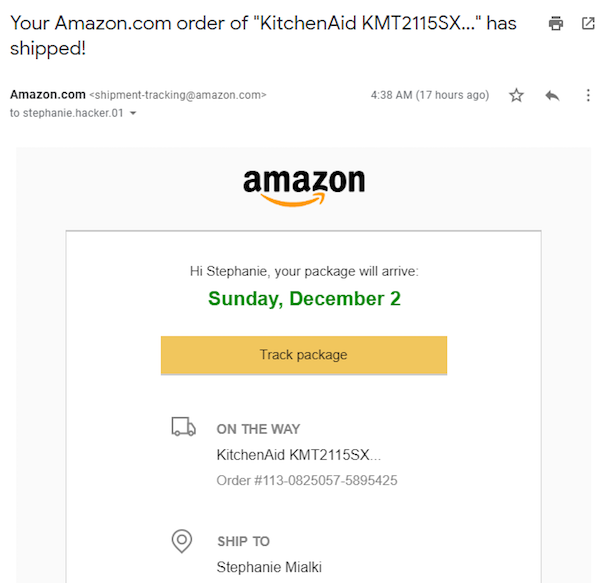This is a digital screenshot from Amazon showing a shipment notification for a user's order. The top of the image displays the message: "Your amazon.com order of KitchenAid KMT-2115SX has shipped," with a small printer icon situated to the right side. Beneath this line, "Amazon.com" is written in bold, black font. 

Further down, there is an email address followed by the directive, "Shipment tracking at Amazon.com." A timestamp indicates the time as 4:38 AM, with "(17 hours ago)" mentioned in parentheses. The recognizable Amazon logo, featuring black text with an orange arrow pointing to the right, is prominently displayed. 

Following this, a personalized greeting reads, "Hi Stephanie, your package will arrive Sunday, December 2nd." An orange "Track Package" button is visible below this message. Accompanying this button is a small truck icon with the text "on the way" next to it. Finally, the order number "113-082-5057-5895425" is listed at the bottom of the screenshot.